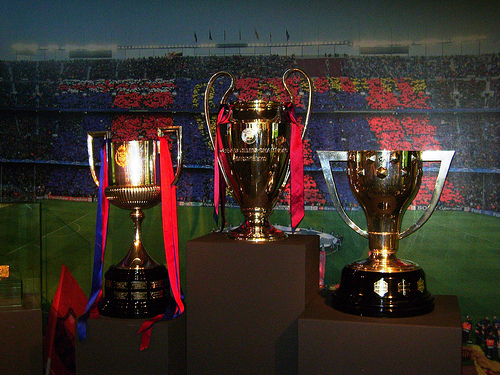The image features a close-up of three gleaming trophies displayed prominently against the vibrant backdrop of a large stadium. The stadium, with a lush green football field, is filled with spectators whose clothing forms vivid waves of red and blue in the stands. The sky above is a clear blue, adding to the atmosphere of the event. 

In the foreground, the three trophies stand on individual podiums of varying heights, symbolizing first, second, and third places. The central trophy, the tallest and most ornate, features elegant handles, a red ribbon, and a lustrous gold color. It is flanked by the second-place trophy on the left, which is a bronze hue, and the third-place trophy on the right, which has silver handles with a bronze base. All three trophies are mounted on sturdy, dark black bases, reflecting light brilliantly.